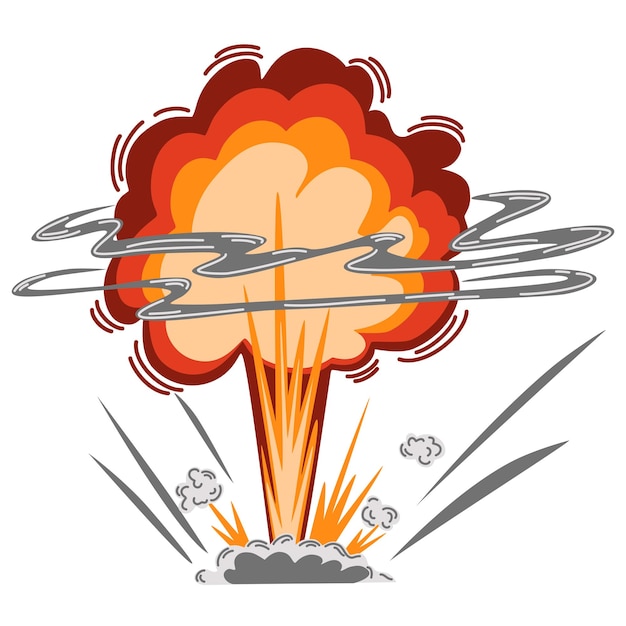This image is a digital cartoonish illustration of a large explosion, likely depicting the impact of a bomb or atomic blast, set against a white background. Central to the image is a dramatic mushroom cloud comprised of various shades of red, orange, and yellow. At the base of the explosion, there is a smaller, dark gray cloud surrounded by lighter gray, almost white, contours. Bursting from the ground level are triangular, sunburst-shaped flames in deeper reds and oranges, transitioning to a yellowish-orange with white highlights. Additional orange and whitish-orange triangular flames emanate from both sides of the mushroom cloud's base.

Rising from the base, the mushroom cloud exhibits a tall column of fiery hues, culminating in a rounded cloud at the top. This upper part of the cloud is accented by thin, double gray lines of smoke swirling around its middle, possibly representing the chaotic movement and intense energy release typical of such explosions. On either side of the central mushroom cloud, there are popcorn-like gray clouds, two on the right and one on the left, adding to the sense of widespread destruction.

Enhancing the sense of movement, there are spiky gray lines forming at 45-degree angles from the base, suggesting waves of shock or debris propelled by the blast. The overall depiction conveys a sense of tremendous impact and energy, marked by the intricate play of colors and shapes symbolizing the explosive force.